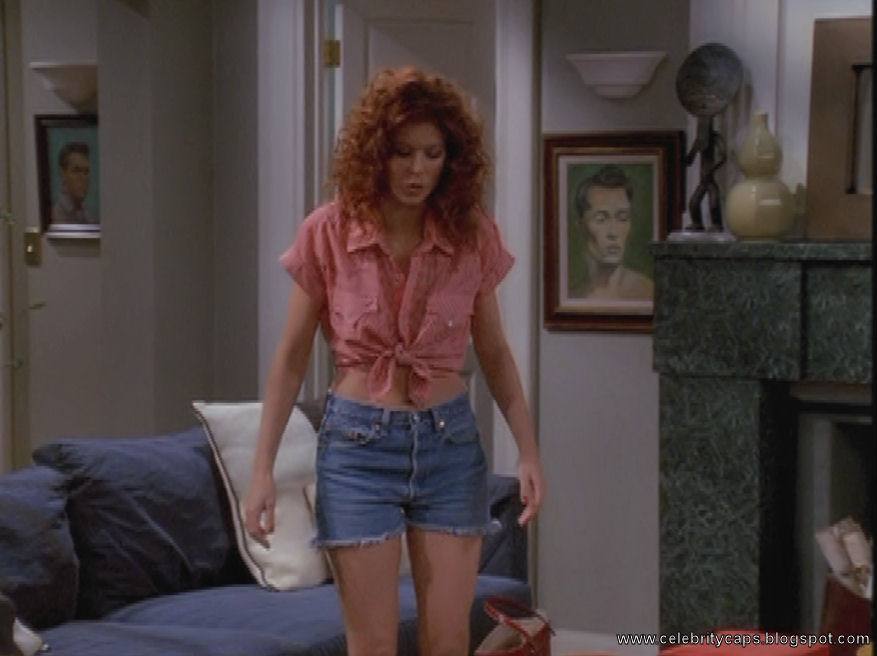In this vibrant scene from "Will & Grace," Deborah Messing, portraying the character Grace Adler, is captured in an apartment living room. Grace, a white actress with striking red hair reminiscent of Annie, is dressed in casual yet stylish attire. She dons a pair of Daisy Duke-style denim shorts that are frayed at the bottom, paired with a pink t-shirt tied above her belly button.

Behind her, a cozy blue couch adorned with a white pillow adds a touch of comfort to the setting. To the right of the frame, a prominent green marbled fireplace catches the eye, with eclectic art pieces sitting on the mantle. Among them, one sculpture resembles a spoon with arms and legs, while another, a white blob-like figure, sits nearby, reminiscent of a headless snowman. Partially cut off at the edge of the photo is a thick-bordered mirror, possibly brown or copper in hue.

On the wall between Grace and the fireplace hangs a portrait of a man, distinct in its colored pencil style. Above this portrait, a light fixture resembling half a teacup adds a quirky touch. In the background, a white-bordered entrance and a white door provide a glimpse into another room. To Grace's left, another similarly styled portrait of a man is visible, with another teacup-like light fixture placed above it.

Grace is looking down at a red purse, open and resting at the bottom center of the photograph, its strap suggesting it's ready for use. The scene captures a moment rich in detail and character, reflective of the show's vibrant aesthetic.